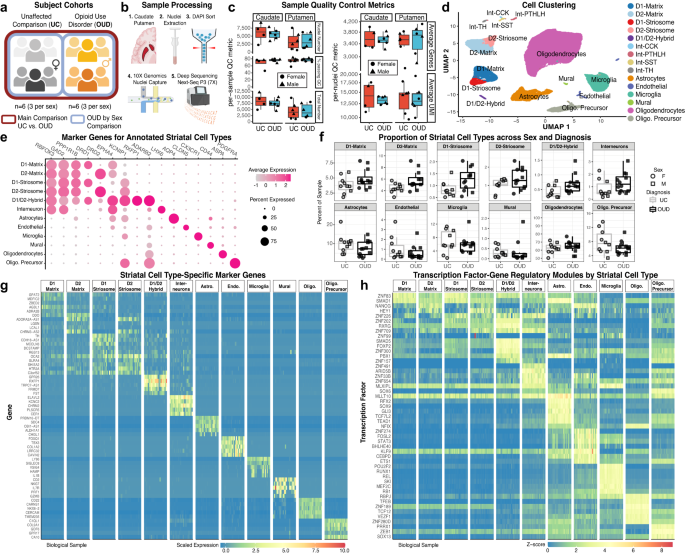This image is a detailed and complex diagram, primarily consisting of multiple graphs and charts that explain various aspects of cell types and their markers. At the top, diagrams A through D highlight different stages and metrics involved in the study: "Subject Cohorts" comparing unaffective comparison and opioid use disorder, "Sample Processing," "Sample Quality Control Metrics" using UC and OUD labels with red and blue rectangles, and "Cell Clustering" presented on a UMAP plot with different colored dots representing clusters.

The second row delves deeper, starting with diagram E, "Marker Genes for Annotated Striatal Cell Types," showcasing a grid with pink and magenta circles indicating expression levels, percent expressed, and average expression. Adjacent is diagram F, "Proportion of Striatal Cell Types Across Sex and Diagnosis," displaying complex shapes in rectangles, with keys identifying sex (female and male) and diagnosis (UC, DUD).

The bottom row presents large bar graphs G and H. Diagram G, "Striatal Cell Type Specific Marker Genes," features bars filled with green to yellow to red squares, marked by gene labels and scaled expression. Diagram H, "Transcription Factor Gene Regulatory Modules by a Striatal Cell Type," utilizes a similar style, indicating transcription factors with a z-score scale. Colors vary across these diagrams from pink, blue, yellow, and magenta, representing different data points, making it a visually intricate representation of medical research focused on cell types.